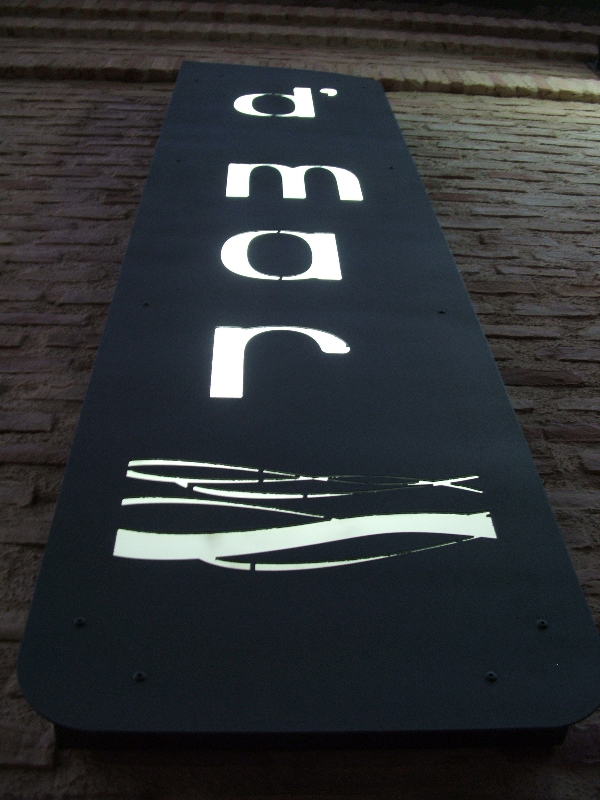This image captures a vertically aligned, rectangular black sign mounted on a brick wall, viewed from a low camera angle looking upward. The prominent white text on the sign reads "D'MAR" with each lowercase letter (d, m, a, r) stacked one below the other, written vertically. The black sign features the letter "D" with an apostrophe next to it at the top, followed by the letters "M," "A," and "R." Beneath these letters, there are intricate white squiggly lines forming a fancy design, including a broad, wavy bar at the bottom. Although the sign is squared off at the top, it has a distinctive rounded bottom and spans the entire height of the image. The brick wall provides a textured backdrop, and the asymmetrical framing adds a dynamic visual tension. There are no people or vehicles present in the scene.